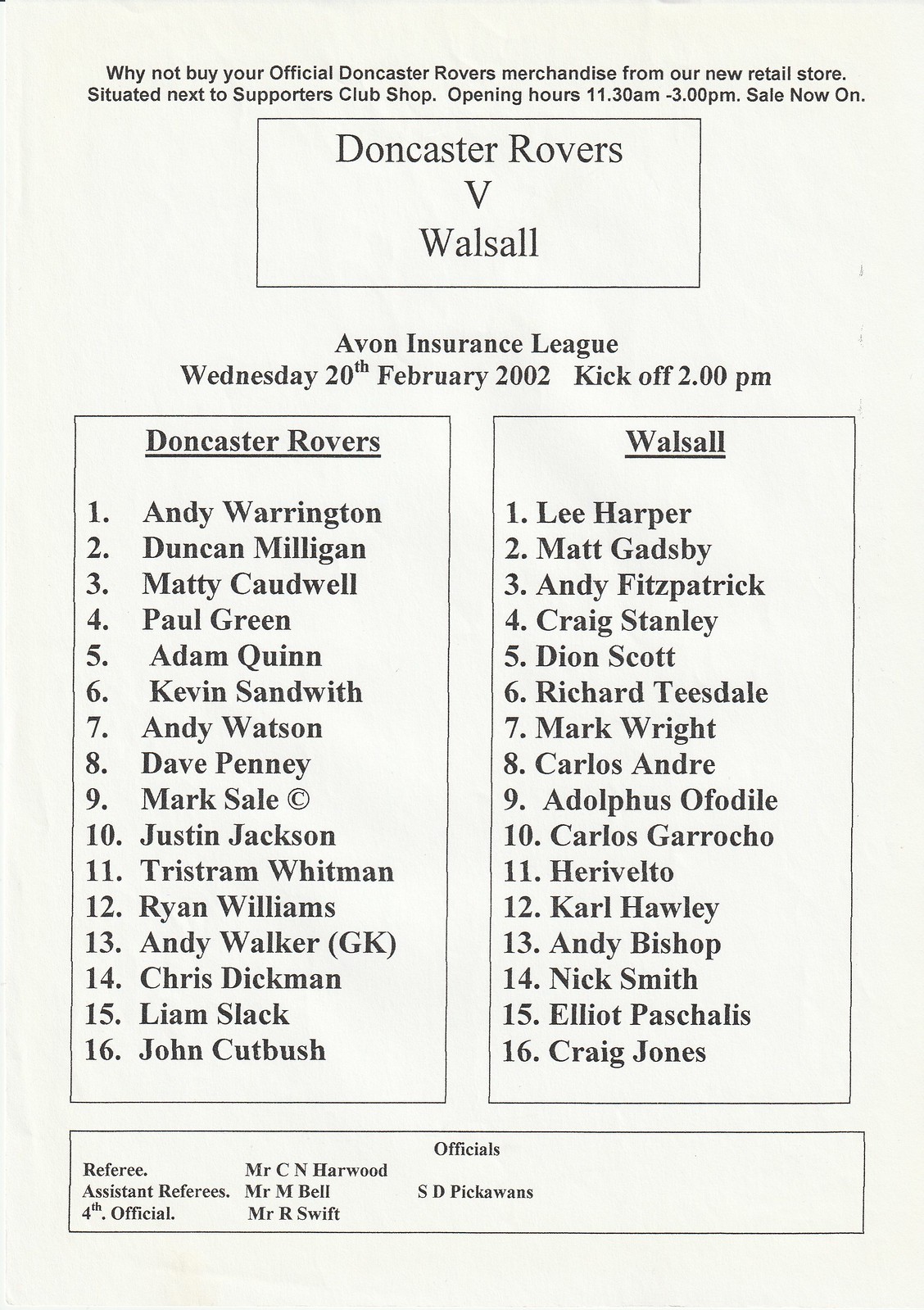This image appears to be a page from a program, featuring text-only content set against a white background with black lettering, indicative of an upcoming soccer game. At the very top, a promotional message urges, "Why not buy your official Doncaster Rovers merchandise from our new retail store," located next to the Supporters Club Shop, and notes the store's opening hours, 11:30 a.m. to 3 p.m., highlighting that a sale is now on. Centrally positioned and enclosed in an outlined box, the text reads, "Doncaster Rovers vs. Walsall," with details for an Avon Insurance League match scheduled for Wednesday, 20th February 2002, with a kickoff at 2 p.m. Below this, two columns delineate the team rosters: Doncaster Rovers on the left and Walsall on the right, each listing players from 1 to 16. Below the team lists, another outlined box details the match officials, including referee Mr. C. N. Howard, assistant referees Mr. M. Bell and S. D. Pickens, and fourth official Mr. R. Swift. The overall layout is well-spaced, and the centered placement of the team names makes them the focal point of the composition.